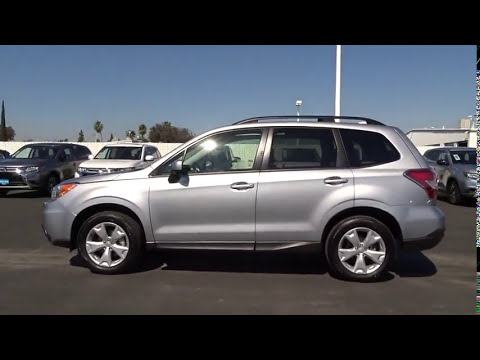This photograph captures an outdoor parking space characterized by a clear blue sky and a gray ground. Dominating the center of the image is a shiny silver SUV, its front facing to the left, possibly in a running state given the reflection of sunlight on the front driver windshield. The SUV is equipped with roof rails, suggesting it is ready for additional transport duties. Surrounding this central vehicle, towards the boundary of the parking lot, are several other parked cars—another silver SUV, a white SUV, and an additional silver SUV. A tall white pole stands behind the central SUV, providing a vertical visual element against the otherwise horizontal expanse. Beyond the boundary fence, one can see the tops of trees and a glimpse of a building, adding depth to the background. The composition is framed by two horizontal black strips at the top and bottom, focusing the viewer’s gaze on the scene within.